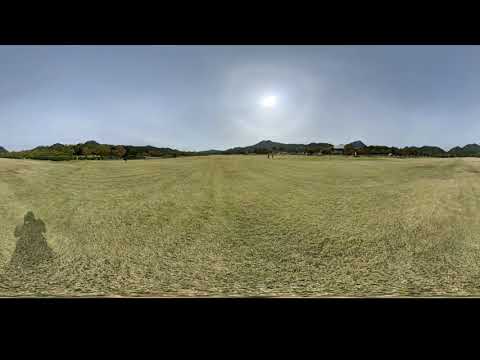The image depicts an expansive, flat, and mostly empty green field, partially bleached as if recently mowed, under a clear blue sky. The sun, positioned near the top of the picture, casts a noticeable white halo that softens its harshness. In the distant background, rough and uneven green hills add depth to the scene, and there appear to be a couple of indistinct figures standing near the center of the image, juxtaposed against these hills. Notably, on the far left side, the shadow of the photographer, possibly resembling a woman in a dress, is visible on the ground. The overall vastness of the field and the wide open sky dominate the frame, while the sun, with its delicate halo, illuminates the serene landscape.